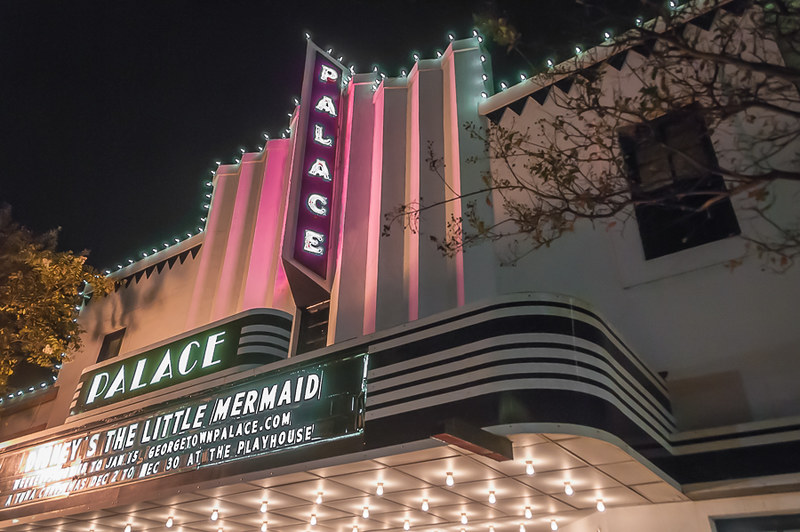This photograph, taken outdoors at night, captures a vintage movie theater known as the Palace. The building, viewed at an angle, is white and adorned with numerous string lights along its roofline, creating a striking silhouette against the dark sky. A prominent vertical sign extends from the center of the building, featuring a pink background with white lights that spell out "Palace". Below this, a horizontal black marquee displays "Palace" in white letters, followed by another black banner indicating the currently showing movie, "Disney’s The Little Mermaid". Additional information on the marquee includes the dates "December 2nd to December 30th at the Playhouse" and "January 15th, GeorgetownPalace.com". The well-lit canopy below the marquee adds to the theater's nostalgic charm, while trees flank the theater on both the left and right sides, framing the scene.